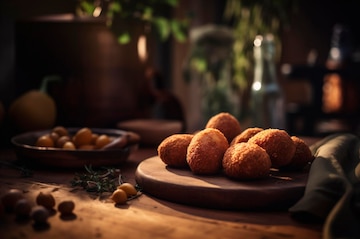In this small, somewhat compressed photograph, the main focus is a wooden platter on a wooden table, showcasing a selection of oval-shaped, golden-brown pastries or dumplings with a textured surface. To the left of the main plate, there is a smaller, slightly out-of-focus wooden bowl filled with what appear to be beans, and there are additional scattered beans on the table in front of the plates. The background of the image, which is out of focus, hints at an indoor setting, possibly a restaurant or kitchen, with some visible plant life, including a pot with green leaves, as well as several glass bottles and other indistinct objects. A ray of sunlight or artificial light illuminates the main plate, adding a touch of warmth to the scene.